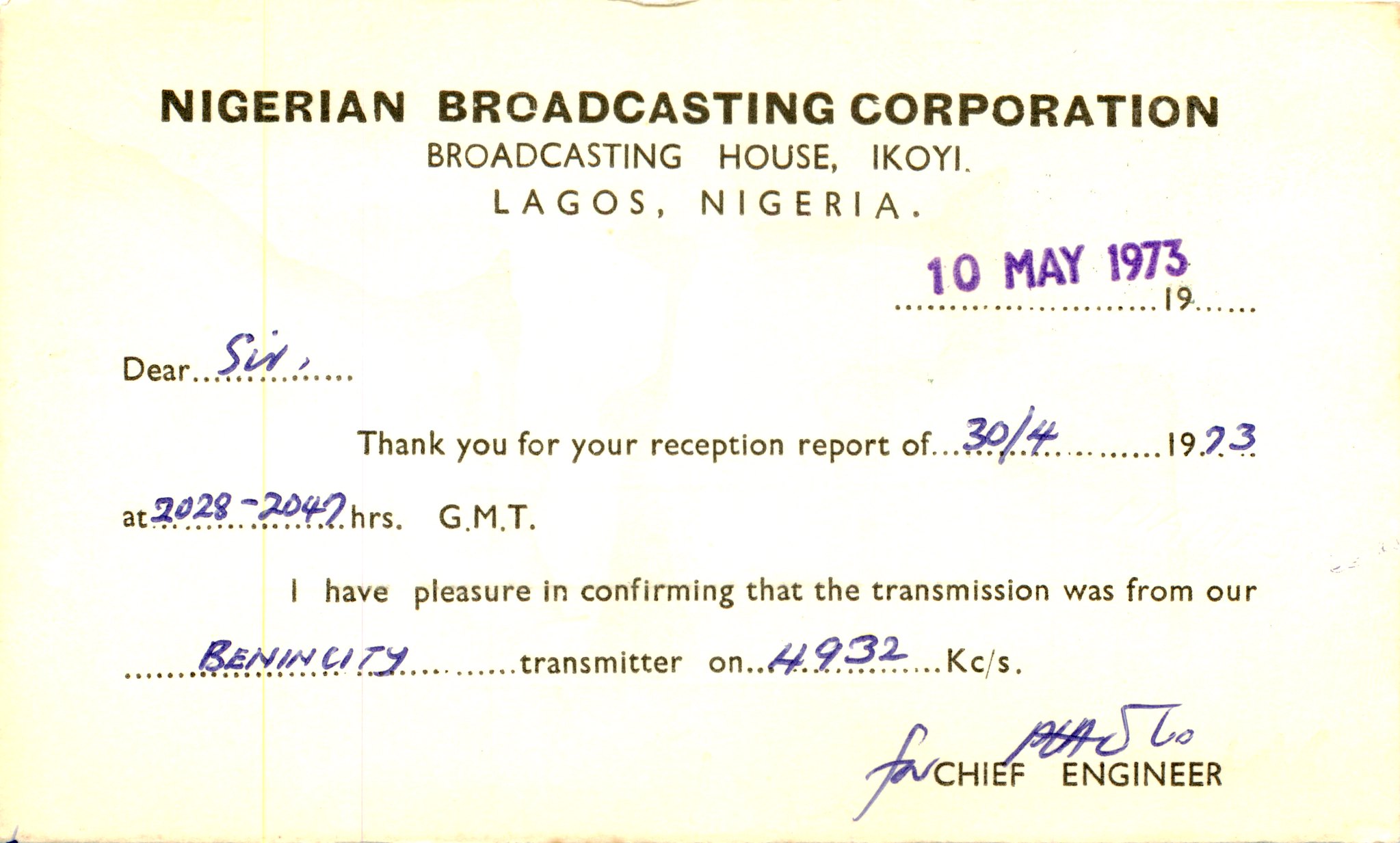The image is a color photograph of a vintage print radio transmission report card in landscape orientation, featuring an aging, yellowed rectangular piece of paper. At the top center, in bold capital typewritten letters, it reads "NIGERIAN BROADCASTING CORPORATION." Below that, in smaller capital letters, it states "BROADCASTING HOUSE, IKOYI." Further down, it says "LAGOS, NIGERIA." To the lower right of this section, a purple date stamp reads "10 MAY 1973."

Handwritten in blue ink to the left, the salutation "Dear Sir" appears below the header. The report continues with pre-typed text followed by handwritten details: "Thank you for your reception report of 30/4/1973 at 2028 to 2047 hours GMT. I have pleasure in confirming that the transmission was from our Benin City transmitter on 4932 KC/S."

The document bears several crease marks, with the edges notably more yellowed than the center. At the bottom right, it is signed by the Chief Engineer in blue ink, though the signature is illegible.